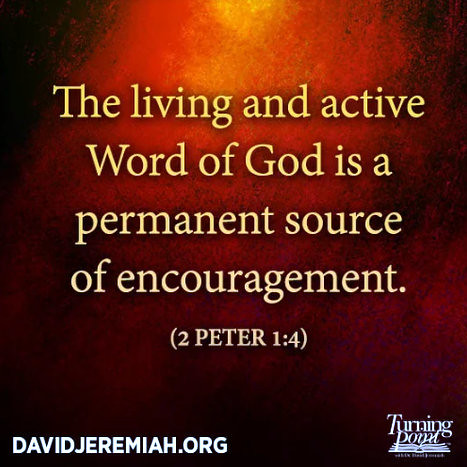This advertisement features a vivid background resembling a swirling blend of red, orange, and dark colors, reminiscent of molten lava or a dramatic sunset. At the very center, prominently displayed in yellow text, is a Bible quote: "The living and active Word of God is a permanent source of encouragement" (2 Peter 1:4). The bottom left corner of the image includes a white watermark with the web address "DavidJeremiah.org." In the bottom right corner, also in white, the text reads "Turning Point" overlaid on an image of an open book, signifying a logo. The overall image is a striking, square-shaped design meant to capture attention and convey a sense of inspiration and faith.